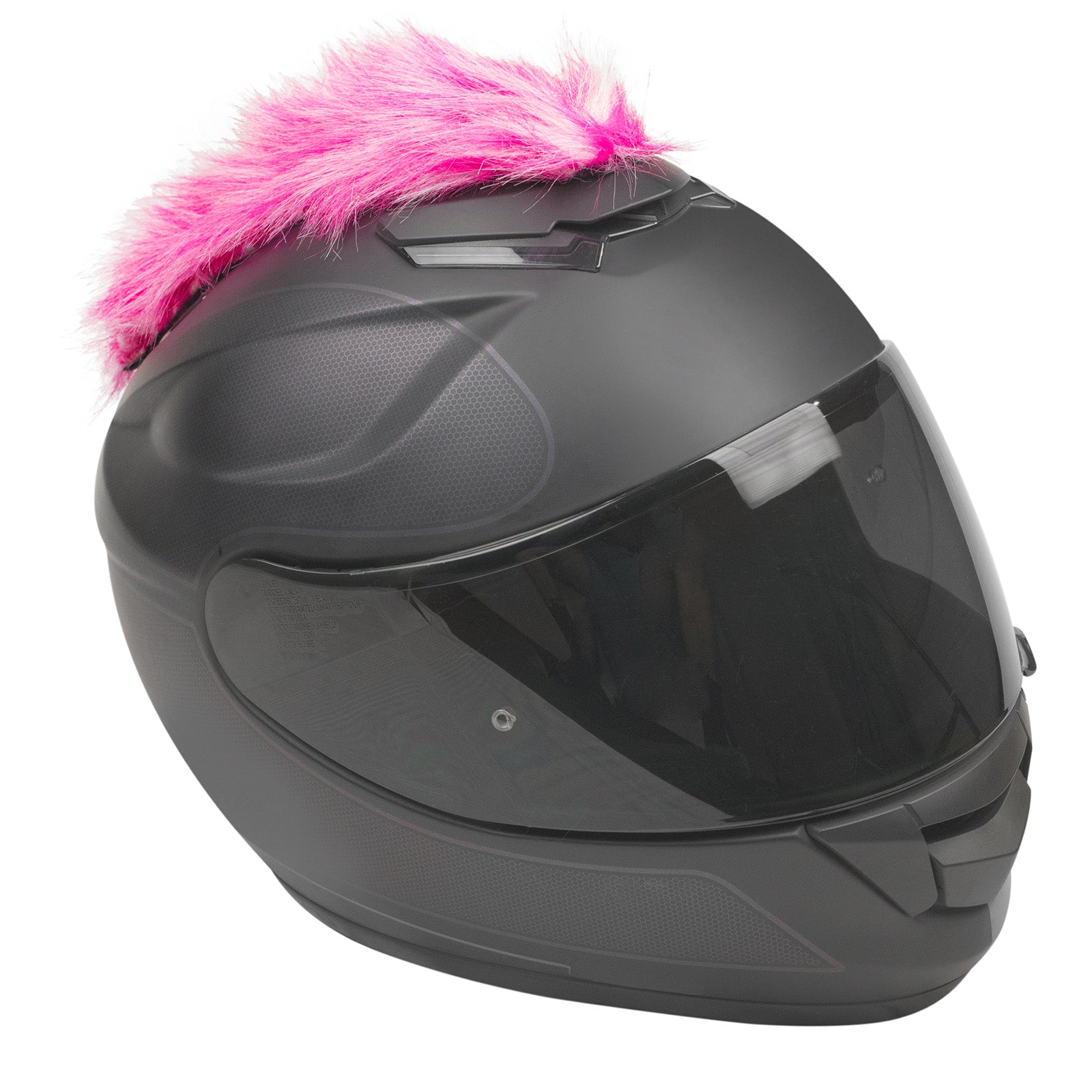The image captures a visually striking, highly detailed photograph of a sleek, all-black motorcycle helmet made of a strong plastic or possibly carbon fiber material, identifiable by its textured surface. The helmet features a darkened, tinted visor to shield the wearer from the sun and boasts an aerodynamic design that tapers to a point in the front before widening towards the rear. Positioned in a three-quarters view with its front pointing slightly left and downward, the helmet's menacing look is boldly contrasted by a vibrant, bright neon pink furry tail attached to the top. This whimsical addition resembles a mohawk that runs from the front to the back, adding a playful touch to the otherwise stark black helmet. The helmet rests against a pristine white background, enhancing the contrast between the dark helmet and the vivid pink tail, making the image both striking and memorable.